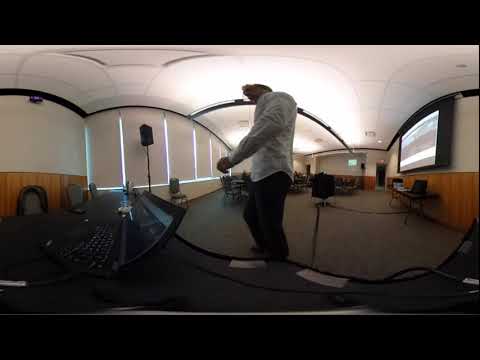The image captures an indoor conference room with a slightly distorted, curved appearance, possibly due to a 360-degree camera. The room features white upper walls and ceilings, while the lower half of the walls have a wooden border. Along the left side, large windows with white drapes partially cover the light. At the center of the image stands a light-skinned man dressed in a white button-down shirt and black slacks. He stands in front of a long black table, which has black tape securing wires onto its surface, and a laptop positioned prominently. Behind the table are several chairs. To the right, there's a projector screen mounted on the wall, with a smaller table below it holding books and various items. The room's floor has gray carpeting, and it's populated with numerous chairs and tables, indicating it is set up for a conference or meeting.